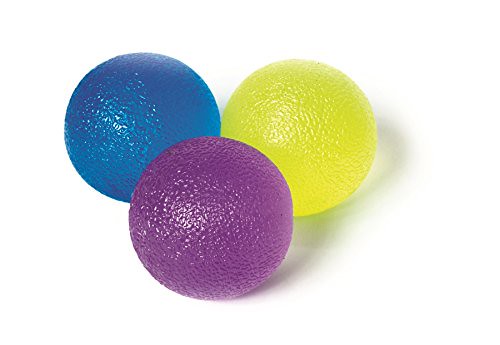This image features three vividly colored balls set against a completely white background, each casting light gray shadows. The balls appear almost as if they could be reflective, with a glossy, slightly bumpy texture hinting at a gumdrop or lemon peel surface. Positioned slightly off-center towards the left of the image, the blue ball is located in the top left corner, the yellow ball – with a texture reminiscent of a lemon – is on the top right, and the glittery purple ball is situated in front of the other two, closer to the viewer. The balls are not touching but are closely spaced, and appear to shimmer with sparkles, showcasing tiny reflective highlights that suggest a light source from the left side of the image.